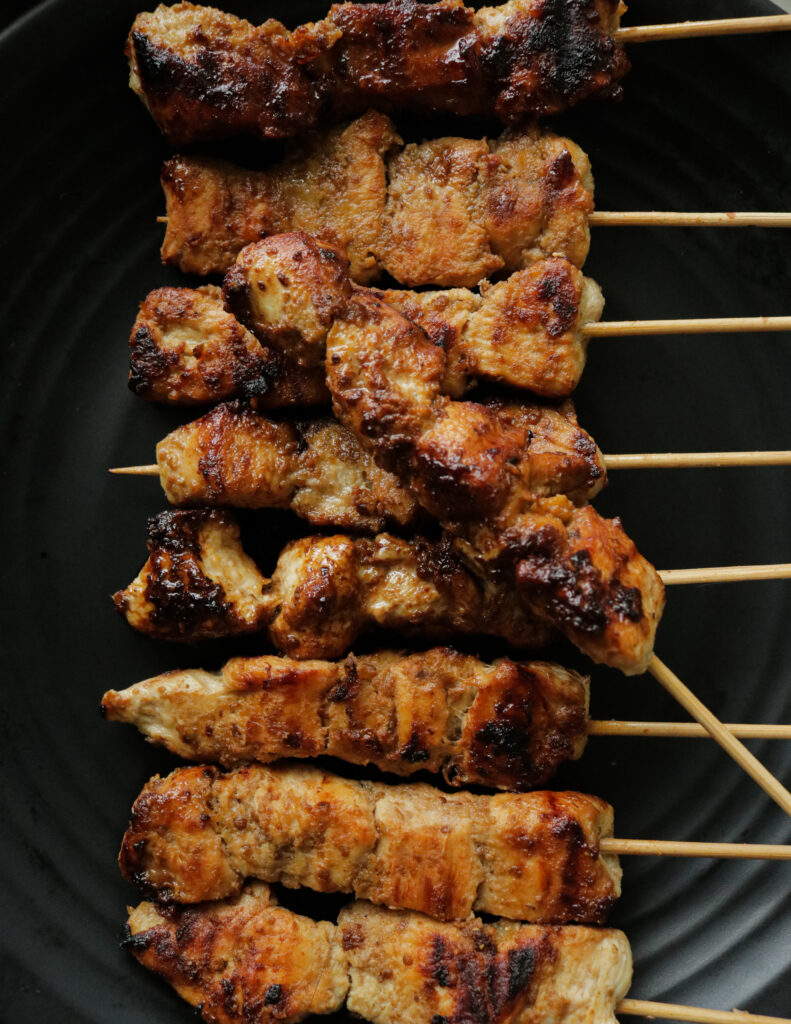The image captures a close-up of nine grilled chicken shish kebabs atop a black, matte-finish plate with concentric ring detailing. Eight of the kebabs are neatly aligned in parallel, while one skewer crosses diagonally over them. Each wooden skewer holds approximately five pieces of cubed chicken, which are charred and appear darker in places, suggesting they were cooked over a grill. The chicken pieces, about one inch each, are glossy and moist, likely having been basted with a light orange-colored sauce. The overall color of the kebabs varies from black and white to tan, depending on the level of charring, giving them a deliciously appetizing look. There seem to be no accompanying vegetables or significant seasoning, but the visual appeal lies in the perfectly grilled, succulent chicken cubes.